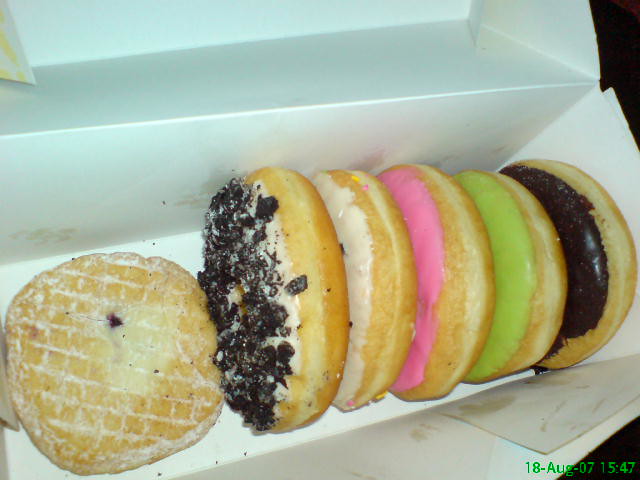This photo, dated August 18, 2007, captures an appetizing assortment of six freshly baked doughnuts arranged in an open white box. The doughnuts display a variety of flavors and toppings, making for a vibrant and delicious sight. On the far left, one doughnut has a jelly-filled center and crisscross patterns of frosting on its tan, baked surface. To its right, a doughnut topped with white frosting is generously sprinkled with Oreo pieces or chocolate crumbles. Continuing to the right, the doughnuts feature a range of colorful frostings: one with creamy white frosting, another with pink frosting, followed by one with a pale green frosting, and finally, a doughnut adorned with chocolate chips. Each doughnut's vivid presentation stands out, enticing viewers with their sweet and appealing exteriors.